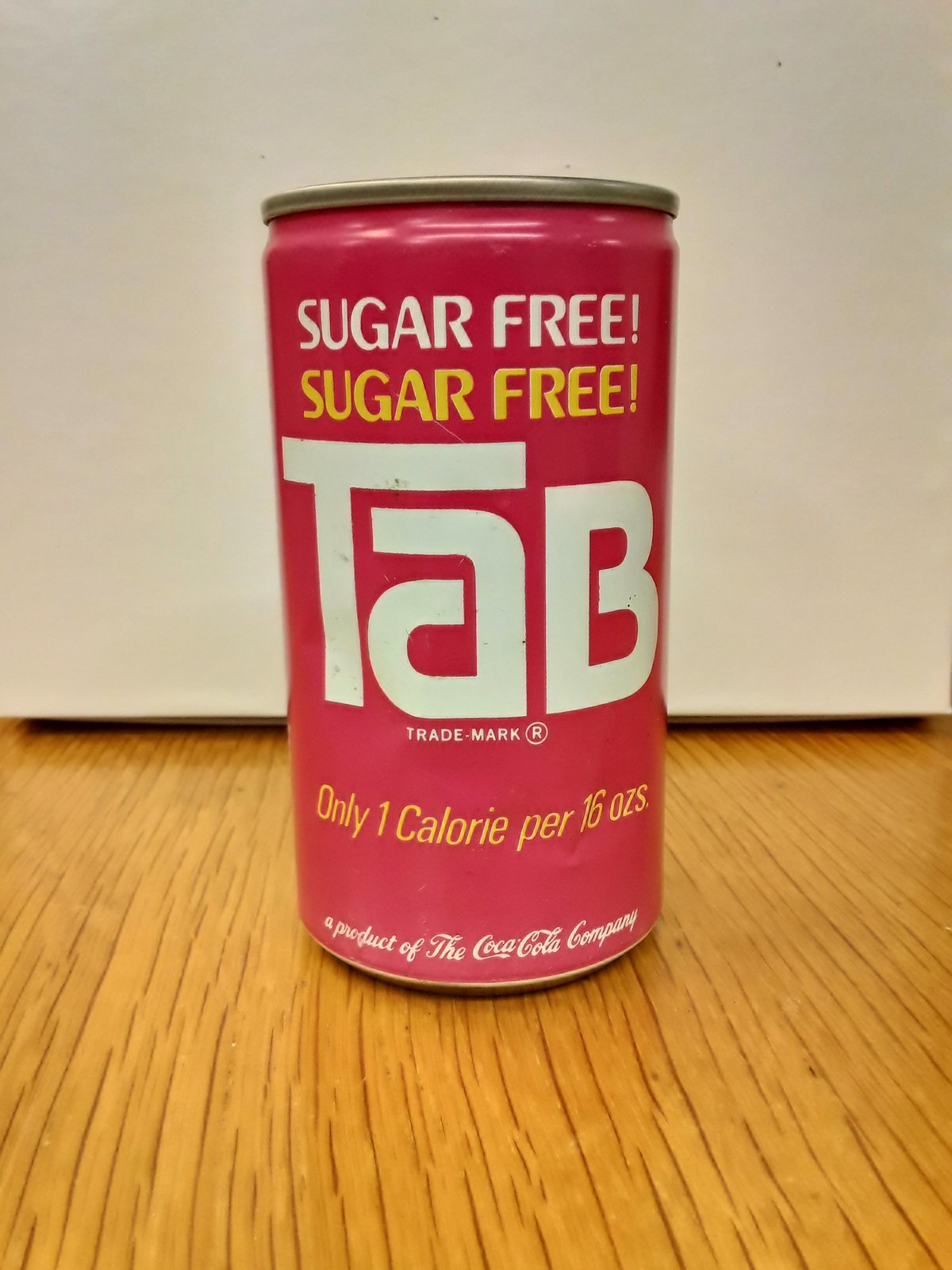The photograph showcases a close-up of a vintage can of Tab, a once-popular sugar-free soft drink. The bright pink, almost magenta can is prominently featured against what appears to be a faux wooden surface, though it could be genuine wood given the peculiar grain and color. The backdrop includes a white element, possibly a wall, appliance, or cabinet, casting a shadow that suggests an unconnected lower edge. The can’s front displays "Sugar-Free" twice—once in white, once in yellow—with an exclamation mark. Below this, the large letters "T-A-B" are written, with a capital 'T' and 'B' and a lowercase 'a,' followed by the registered trademark symbol. It also states in yellow text, "Only one calorie per 16 ounces," and in a cursive-like white font along the bottom rim, "A product of the Coca-Cola company." The can is clearly aged, evident by its dented body, rusted top and bottom, and discolored silver cap, with chipped paint and dirt marks around the emblematic logo.